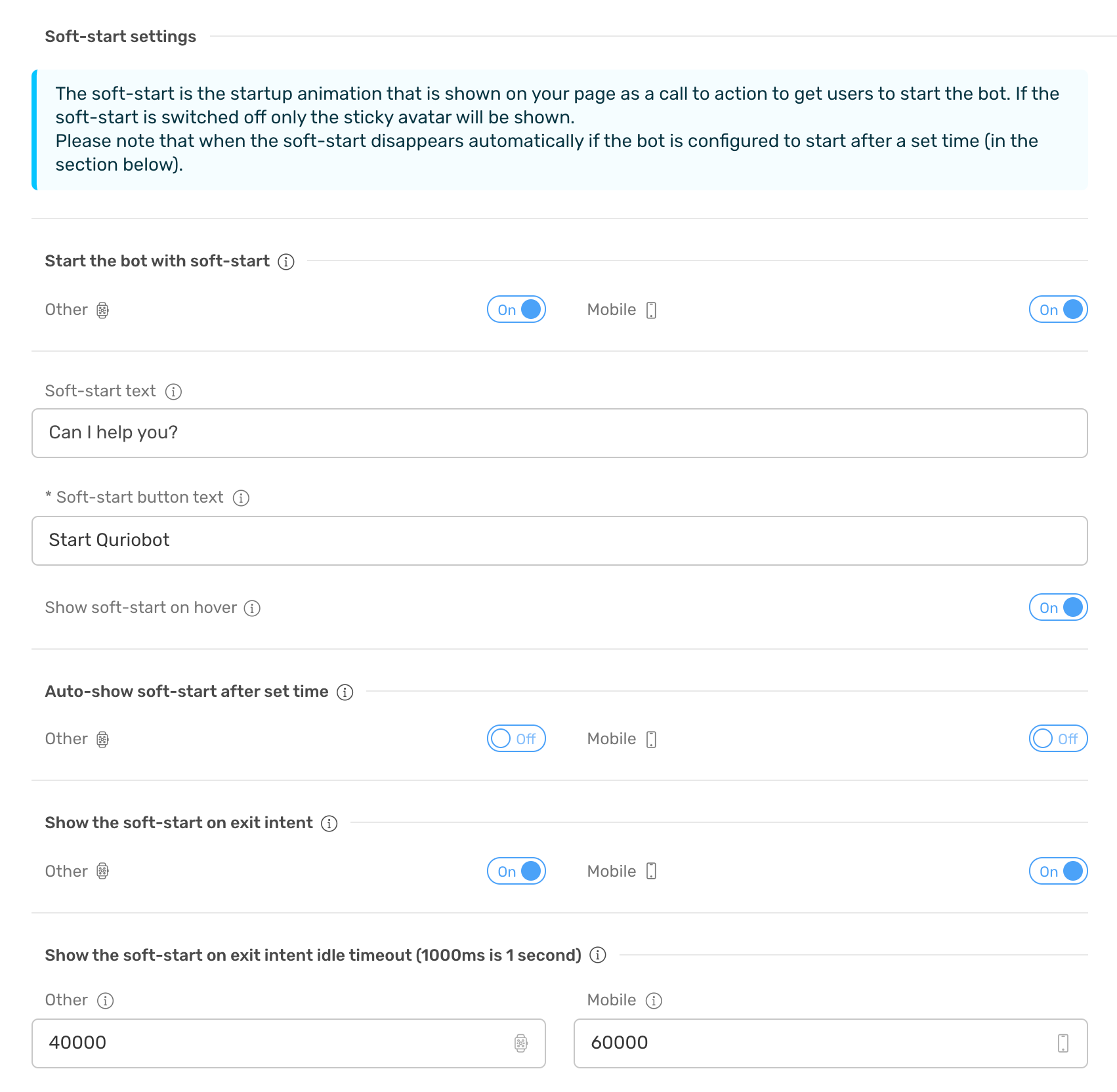This image displays the Soft Start Settings page for configuring the startup animation of a chatbot on a user's webpage. The top section features a light blue banner with a darker aqua blue border on the left side, containing a paragraph that explains: "The soft start is a startup animation shown on your page as a call to action to encourage users to start the bot. If the soft start is switched off, only the sticky avatar will be shown. Please note that the soft start automatically disappears if the bot is configured to start at a set time in the section below."

Below this, there is a section labeled "Start the Bot with Soft Start," accompanied by an information icon ('i' within a circle). The next section, titled "Other," includes a toggle for mobile devices, which is currently switched on. A thin line separates this from the "Soft Start Text" field, which currently contains, "Can I help you?"

Further down is the "Soft Start Button Text" field where "Start Querio Bot" is displayed. There is also an option labeled "Show Start on Hover," which is toggled on. Another line separates this from the "Auto Show Soft Start" and "Set Time" sections, which include options to toggle on "Other" and "Mobile." An additional toggle option is provided to "Show Soft Start on Exit Intent," which is also switched on.

Finally, the settings page includes options to "Show Soft Start on Exit Intent Idle Timeout," with configuration fields for "Other" set to 40,000 milliseconds and "Mobile" set to 60,000 milliseconds.